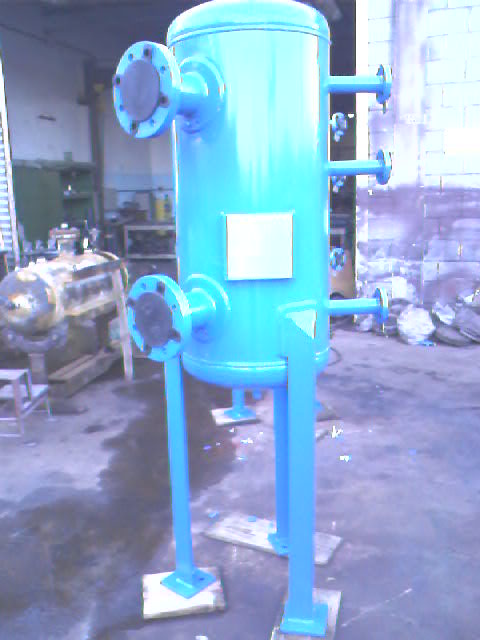The photograph captures a tall, cylindrical blue tank with three legs, positioned in front of a garage or warehouse with a large open bay door. The blue tank sits on wooden planks placed on wet cement. The tank features several knobs, dials, and protruding pipes, all capped and matching the blue color of the tank. There is also a small, white, square sign on the tank, devoid of any writing. The background reveals a brick wall with dirt accumulation near the bottom, and various items scattered on the ground. Additionally, a silver cylindrical object lies on its side with a bench positioned nearby. Inside the open bay door, shelves are visible, and there is a mix of machinery and a workbench to the left. The overall scene appears slightly blurry and overexposed, adding to the industrial, cluttered ambiance of the setting.